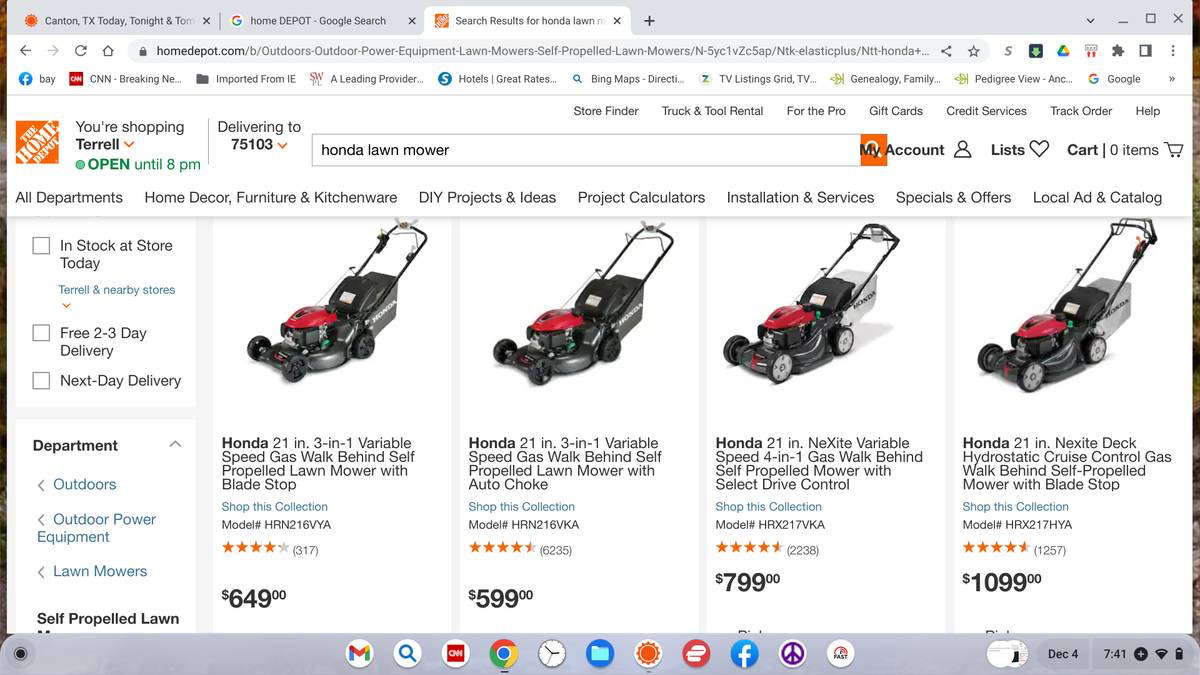A detailed screenshot captures a desktop view of a Chrome browser window with three open tabs. The far-left tab, inactive, displays "Canon Texas today, tonight, and tomorrow," presumably a weather application. The middle tab is dedicated to a Google search about Home Depot. The rightmost and active tab reveals the search results for "Honda lawnmower" on the Home Depot website, specifying the user’s location as zip code 75103 in Terrell, Texas.

In the search bar of the Home Depot website, the query "Honda lawnmower" is prominent. Consequently, the screen showcases four distinct Honda lawnmower models, each displayed horizontally with corresponding images, descriptions, and prices ranging from $649 to $1,099.

1. **Honda 21-inch 3-in-1 Variable Speed Gas Walk-Behind Self-Propelled Lawnmower with Blade Stop**: This model features a blade stop system, has a price tag of $649, and is rated 4 out of 5 stars based on 317 reviews.
   
2. **Honda 21-inch 3-in-1 Variable Speed Gas Walk-Behind Self-Propelled Lawnmower with Auto Choke**: Offering an auto choke system, this lawnmower is priced at $699 and boasts a superior rating of 4.5 stars from 6,235 reviews.

3. **Honda 21-inch NEXITE 4-in-1 Variable Speed Gas Walk-Behind Self-Propelled Mower with Select Drive Control**: This model features the NEXITE deck and Select Drive Control, priced at $799. It has earned a 4.5-star rating from 2,238 reviews.

4. **Honda 21-inch NEXITE Deck Hydrostatic Cruise Control Gas Walk-Behind Self-Propelled Mower with Blade Stop**: The premium model includes hydrostatic cruise control and a blade stop system, priced at $1,099, and it holds a 4.5-star rating from 1,257 reviews.

Each product listing includes the respective features, model numbers, and customer ratings, providing a comprehensive comparison for the potential buyer.